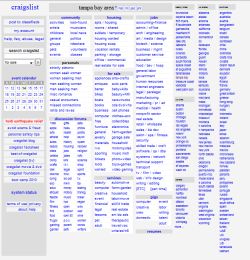This is a blurry screenshot of the Craigslist website, specifically the Tampa Bay area page. The page features a light grey background with "Craigslist" written in blue font at the top left-hand side. In the center of the page, on a slightly darker grey background, the text "Tampa Bay area" is displayed in black font. The rest of the page consists of various headers and categories, predominantly formatted in blue text on a very light grey, almost white, background.

At the top of the list, there are headers like "community" followed by what appears to be "booking" or "banking," then "jobs." In the next row, there are headers for "for sale" and "discussions," followed by "services," and at the bottom, "gigs." Each header has subcategories listed beneath them, but they are too small to decipher due to the blurriness.

On the left-hand side, under the "Craigslist" title, there are several header options including "something," "my account," and another unclear header. Below these, there is a search function with a white text window and a drop-down menu currently set to "for sale," along with a search button. Beneath the search bar is a calendar, followed by some unreadable red text, and then another list in blue.

Despite the blurry quality of the photo, it is evident that this page belongs to the Craigslist Tampa Bay area.